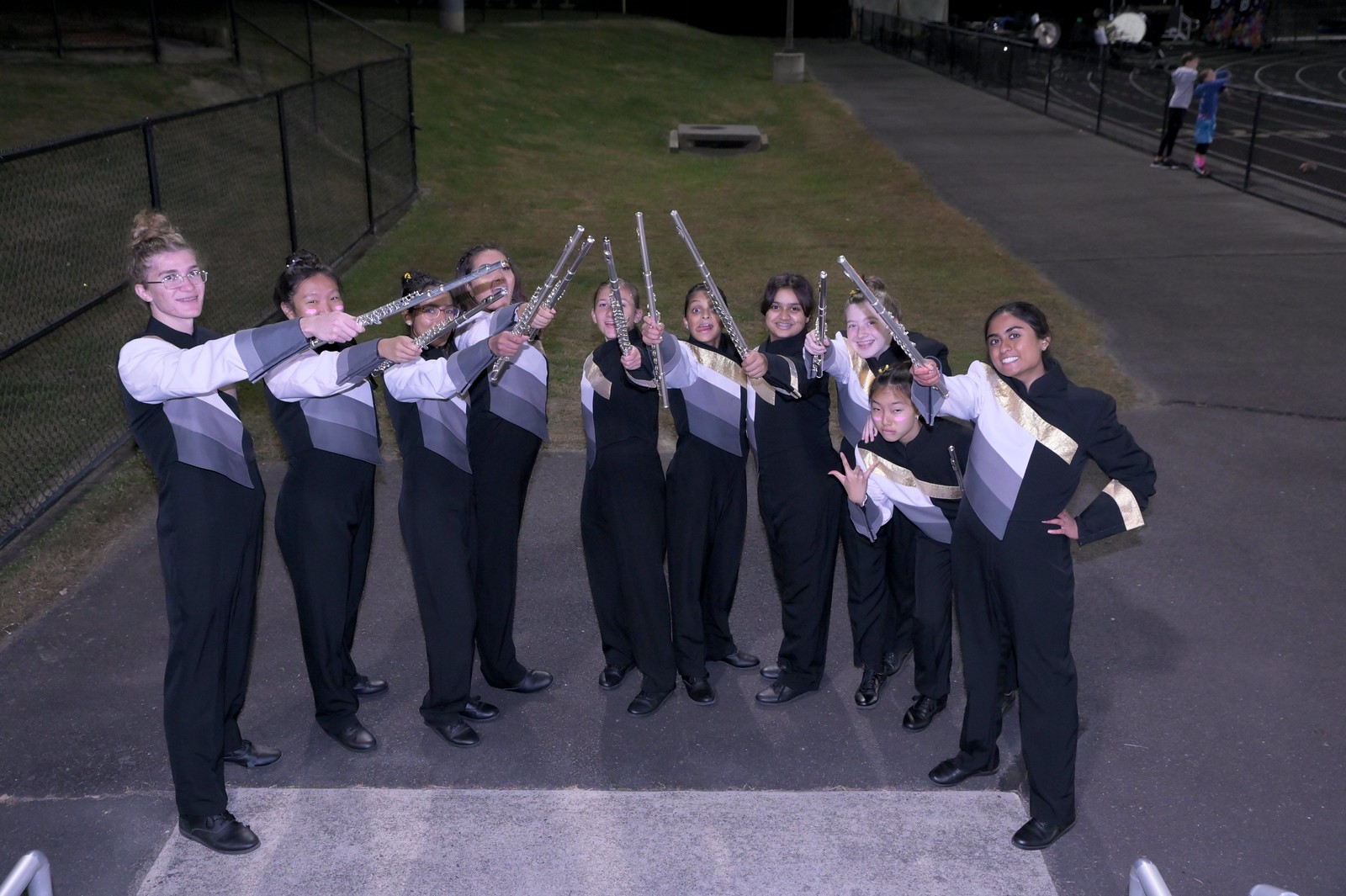In this photo, we see a group of school band members, appearing to be high school students, arranged in a semi-circular formation. The group is composed of approximately ten young individuals, encompassing a diverse mix of genders and races, primarily in their teens to early twenties. They are all uniformly dressed, wearing black pants paired with long-sleeve shirts that are designed with a mix of dark gray, light gray, white, and gold stripes, creating a chevron pattern on the front. Notably, one sleeve of each shirt is white while the other is black. They all sport black shoes.

Every member is holding a silver flute-like instrument aloft, pointed towards the center, as if in celebration or forming a unified pinnacle. Interestingly, all the instruments are held in the right hand except for one member who is making a V sign with her left hand.

The setting appears to be an outdoor area with a gray sidewalk, with expansive lawn areas and black fences visible in the background. On the right side of the image, there is a high school running track with a couple of individuals leaning against the fence, observing the scene. The image captures the essence of youthful exuberance and collective pride, possibly after a victory or performance. The lighting suggests that the photo was likely taken towards the evening.